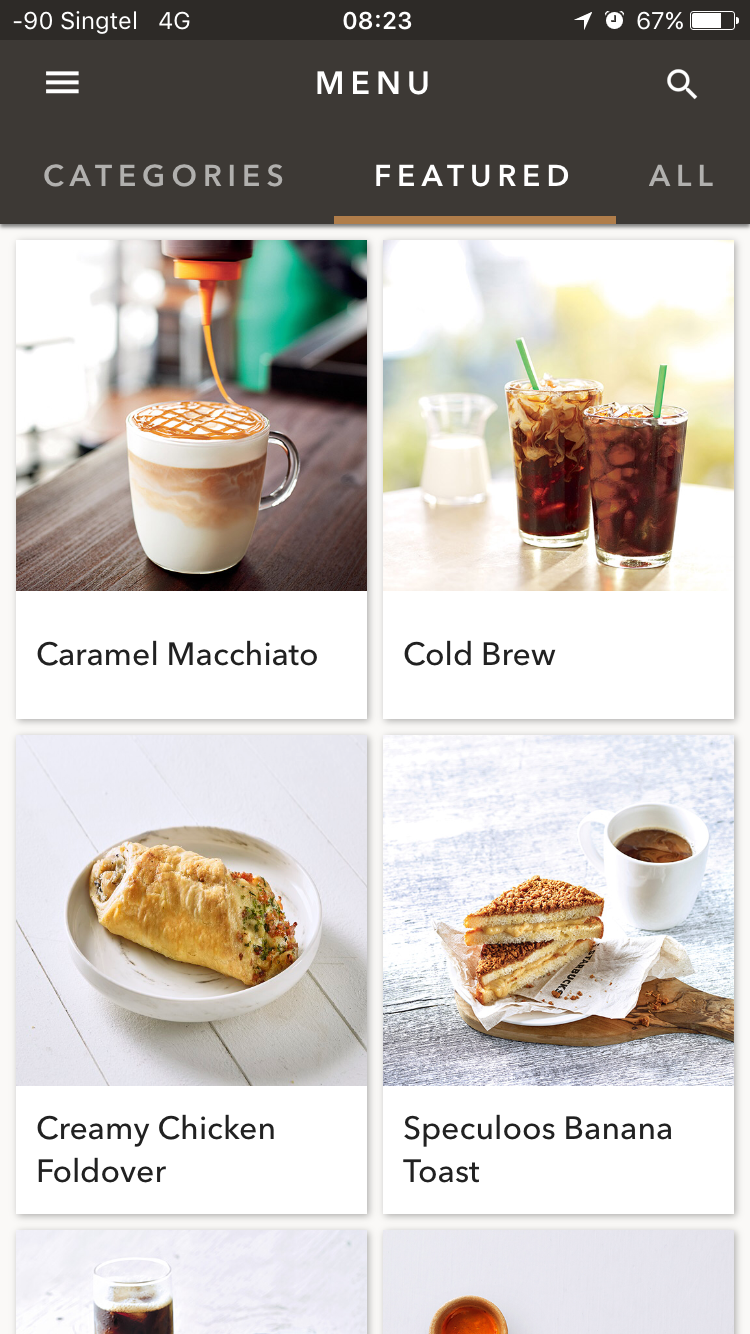A screenshot of a phone displaying a restaurant menu is shown. At the top of the screen, the phone's taskbar indicates a signal of -90 with the carrier SingTel 4G. The time is displayed as 8:23. There are several icons visible including a location icon, an alarm clock, a battery status of 67% with the battery icon filled with white, and an icon with three horizontal lines stacked (likely the menu or info icon). The word "MENU" is prominently displayed in white capital letters against a dark background.

Below the header, a search bar is visible, followed by three options: "Categories", "Featured", and "All". "Featured" is highlighted with bold text and a brown underline, while "Categories" and "All" are in a light gray font.

The featured menu items showcased include:
- A Caramel Macchiato, depicted as two glasses with green straws, looking particularly delicious.
- A Cold Brew, also shown elegantly beside the Caramel Macchiato.
- A Creamy Chicken Fold-over, described as tan and baked beautifully, appearing very appetizing.
- Speculoos Banana Toast, which looks equally enticing.

Some of the other menu items are cut off from the view, but the visible ones are showcased attractively and hint at a delectable dining experience.